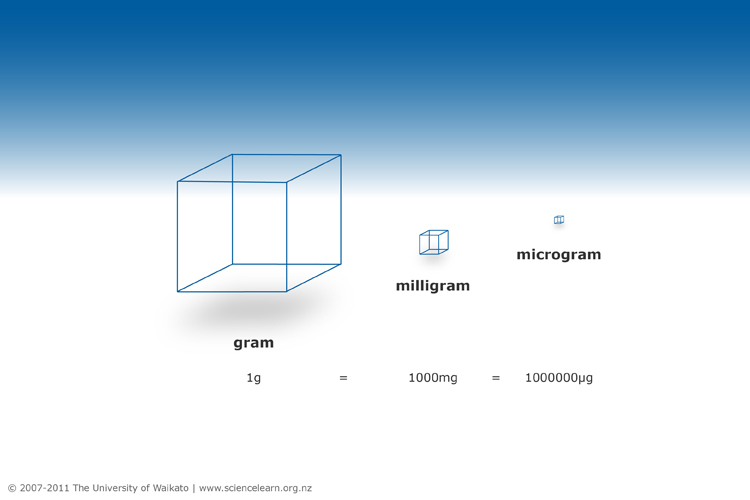The informational image displays the size difference between units of measurement on a background that transitions from blue at the top to white at the bottom. Positioned in the middle are three 3D cubes representing grams, milligrams, and micrograms. The largest cube on the left is labeled "gram" and underneath, it states "1 gram." Next to it, the medium-sized cube is labeled "milligram" with "1,000 milligrams" written underneath. The smallest cube on the right is labeled "microgram," and it notes "1,000,000 µg" (micrograms). At the bottom left of the image, there is a watermark reading, "© 2007 to 2011, the University of Waikato," followed by the website "www.sciencelearn.org.nz".